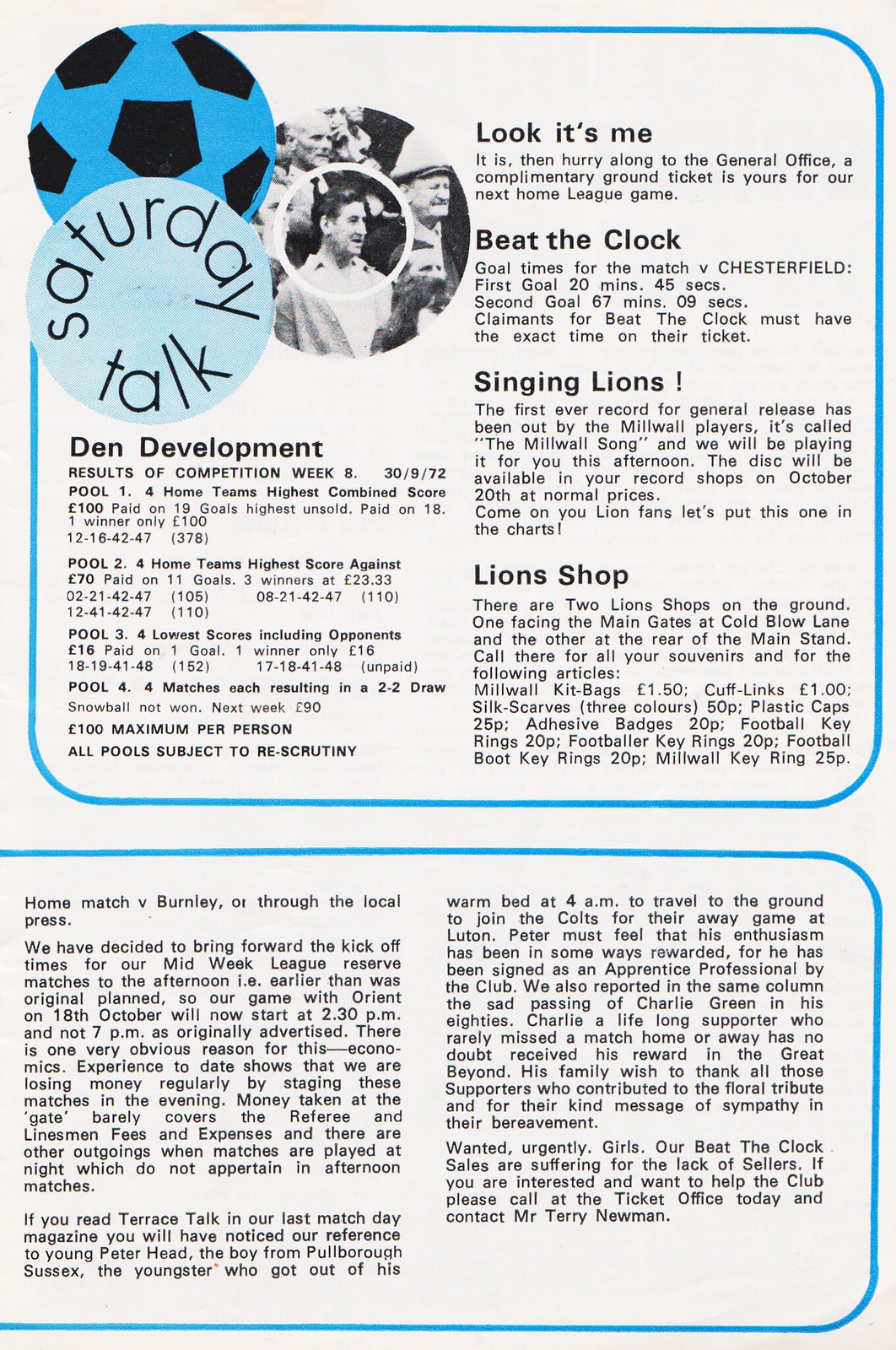This image appears to be a detailed, page-long article from a newspaper or magazine, predominantly in black and white with blue accents. The background is white and adorned with a light blue border. In the top left corner, a blue and black soccer ball is featured next to a blue circle with the text "Saturday Talk" inside. Below this, "DEN Development, Results of Competition Week" is prominently displayed in bold black lettering. The article further details sections labeled as Pool 1, Pool 2, and Pool 3, while noting that "All Pools Subject to Rescrutiny." On the right side of the article, additional sections titled "Look It's Me," "Beat the Clock," "Singing Lions," and "Lion Shop" are arranged sequentially, each followed by corresponding text. A noteworthy element is a black and white photograph of two gentlemen, with one individual's head circled in white, potentially indicating the author or a key subject. The entire layout, characterized by its organized columns and sections, is augmented by blue bordering, giving it a structured and aesthetically pleasing appearance.